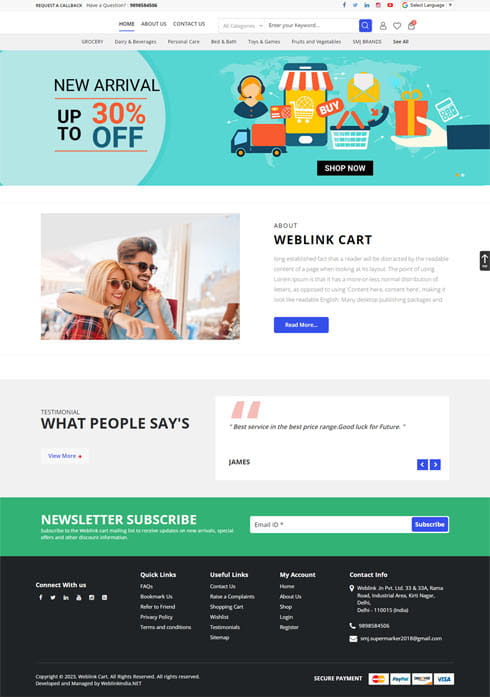Screenshot of a website's homepage features a structured layout with multiple sections. At the very top, there's a slim gray bar populated with small, indiscernible black text on the left, and a collection of social media icons (Facebook, Twitter, Instagram, YouTube, and an unidentified one) on the right. Adjacent to these icons, there's a drop-down menu labeled "Select Language."

Beneath this, a white navigation bar spans the width of the page, starting with the links "Home," "About Us," and "Contact Us" aligned to the left. A search field dominates the center of the bar, flanked by a drop-down menu titled "All Categories" on the left, and containing the placeholder text "Enter Your Keyword" in black font. To the right of this field is a blue square button featuring a white magnifying glass icon, indicating the search function.

Further right on the navigation bar, there are three small icons: a silhouette representing a user account, a heart for favorites or wishlist, and a shopping bag marked with a red circular badge displaying the number "0" in its upper right corner.

Below the main navigation bar is another gray bar with black text, partially legible with categories like "Grocery," "Personal Care," "Bed and Bath," "Toys and Games," and other less readable sections.

Finally, the central area of the page is occupied by a graphic-rich rectangle featuring colorful, cartoon-style illustrations related to shopping, including an image of a delivery truck, a woman wearing a headset indicative of customer service, and various gift items.